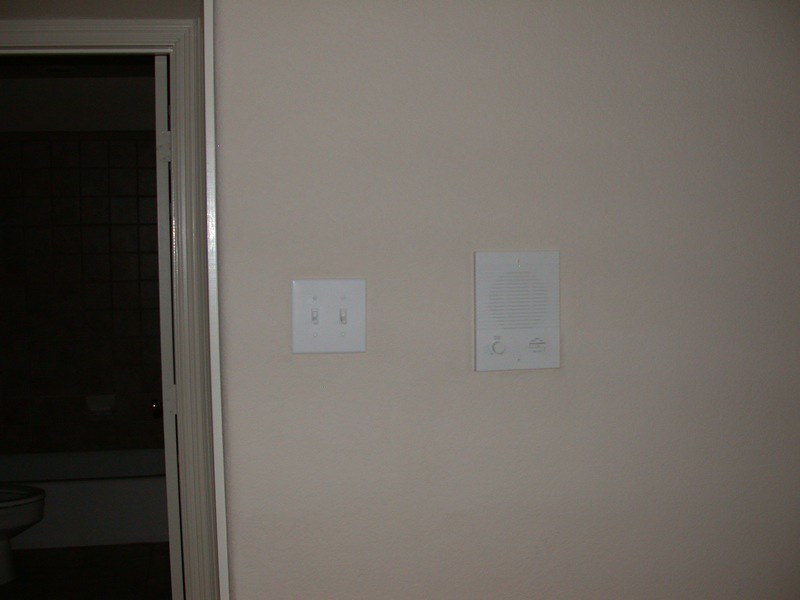The image features a segment of a light brown-painted wall adorned with a white light switch that has two toggles. Approximately six inches to the right of the switch, a white, wall-encased speaker is visible, equipped with a volume knob and a push button for speaking into the integrated microphone. The wall forms part of a scene that slightly opens into a dimly lit bathroom. Through the doorway, part of the bathroom reveals a white bathtub and toilet. The bathtub's surrounding wall is covered in brown tiles, within which a ceramic soap dish is mounted.